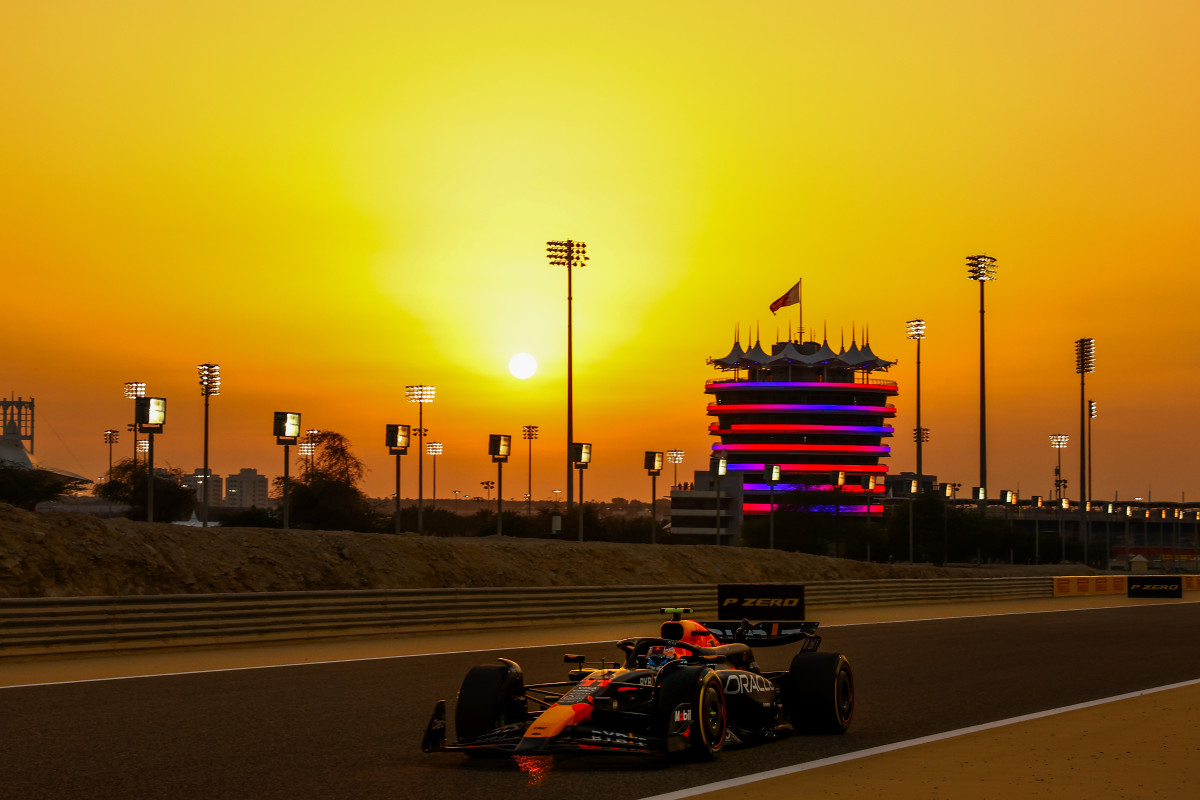The image captures a vibrant scene at an auto raceway during what appears to be either sunset or dawn, as the sky is painted with bright hues of yellow and orange at the horizon, transitioning smoothly into darker shades above due to clouds. The racetrack is lit by a series of stadium lights, casting a glow on the entire area. A modern Formula One car, characterized by its sleek design, large black tires, and a prominent orange stripe down its center with "Oracle" written in white lettering, is positioned on the track, heading towards the left side of the image. The foreground is dominated by the smooth, well-maintained surface of the track, marked by clear lines and concrete barriers.

In the background, a striking multi-level racing tower stands tall, adorned with vibrant red and blue neon lights that encircle its structure. The tower, which features a flag at its pinnacle, offers an unusual appearance with elements that resemble a carousel at the top, adding to the eclectic mix of colors and shapes. The entire setting is bathed in the soft yet vivid light of the setting or rising sun, with no people visible, highlighting the solitude and readiness of the scene for an exciting race event.